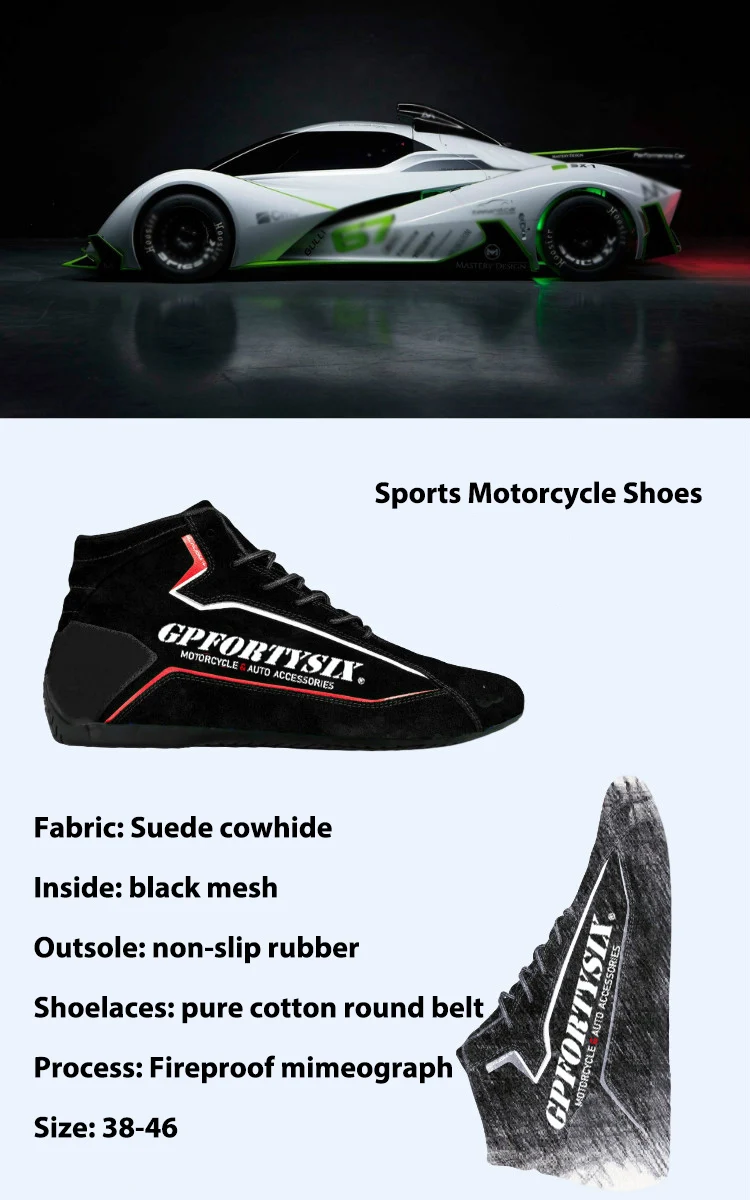The image is a composition of two distinct but related pictures connected by a sports theme. The top picture features a sleek, aerodynamic, white racing car with green details and the number 67 prominently displayed in green. The car has black wheels and lights that have a yellow tint. The backdrop of this image is entirely black, emphasizing the car's refined and futuristic design, which some suggest looks AI-generated. Below this is an advertisement for sports motorcycle shoes, displayed against a blue background. The primary shoe in the ad is black with red and white highlights, prominently labeled with "GP4-46" and detailed descriptions such as "motorcycle and auto accessories." Specific features include fabric suede cowhide interior, black mesh outsole, non-slip rubber, pure cotton round belt shoelaces, and a fireproof mimeograph process. The sizes range from 38 to 46. To the bottom right, there’s an illustration of the shoe, presented vertically with the toe facing upwards, adding a dynamic visual element to the ad. Despite the pairing of a racing car and motorcycle shoes, the cohesive sports theme ties the images together.